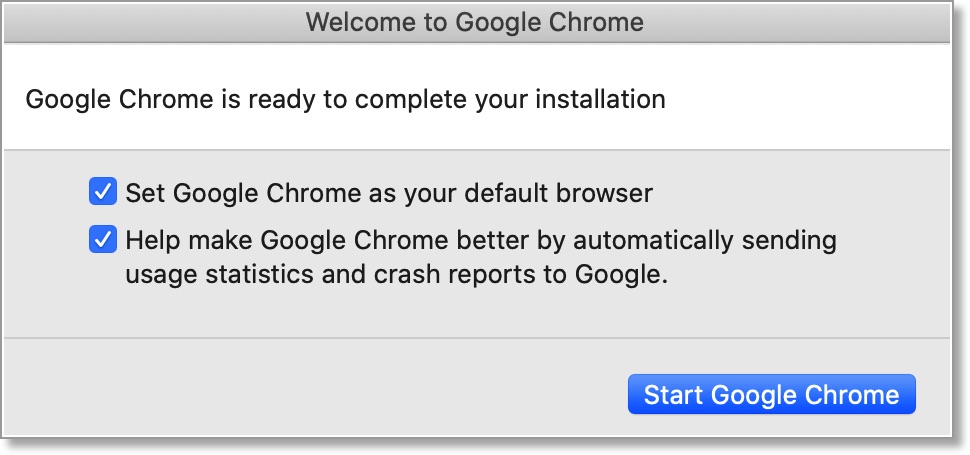A pop-up window from an old version of Google Chrome is displayed. The interface features a gray banner at the top with the text "Welcome to Google Chrome." Below this banner is a white section that reads, "Google Chrome is ready to complete your installation." Underneath, there is a lighter gray area with two blue checkboxes. The first checkbox is labeled "Set Google Chrome as your default browser," while the second reads, "Help make Google Chrome better by automatically sending usage statistics and crash reports to Google." Both boxes are checked by default, but users can uncheck them to customize their installation preferences. At the bottom of the pop-up is a blue button labeled "Start Google Chrome."